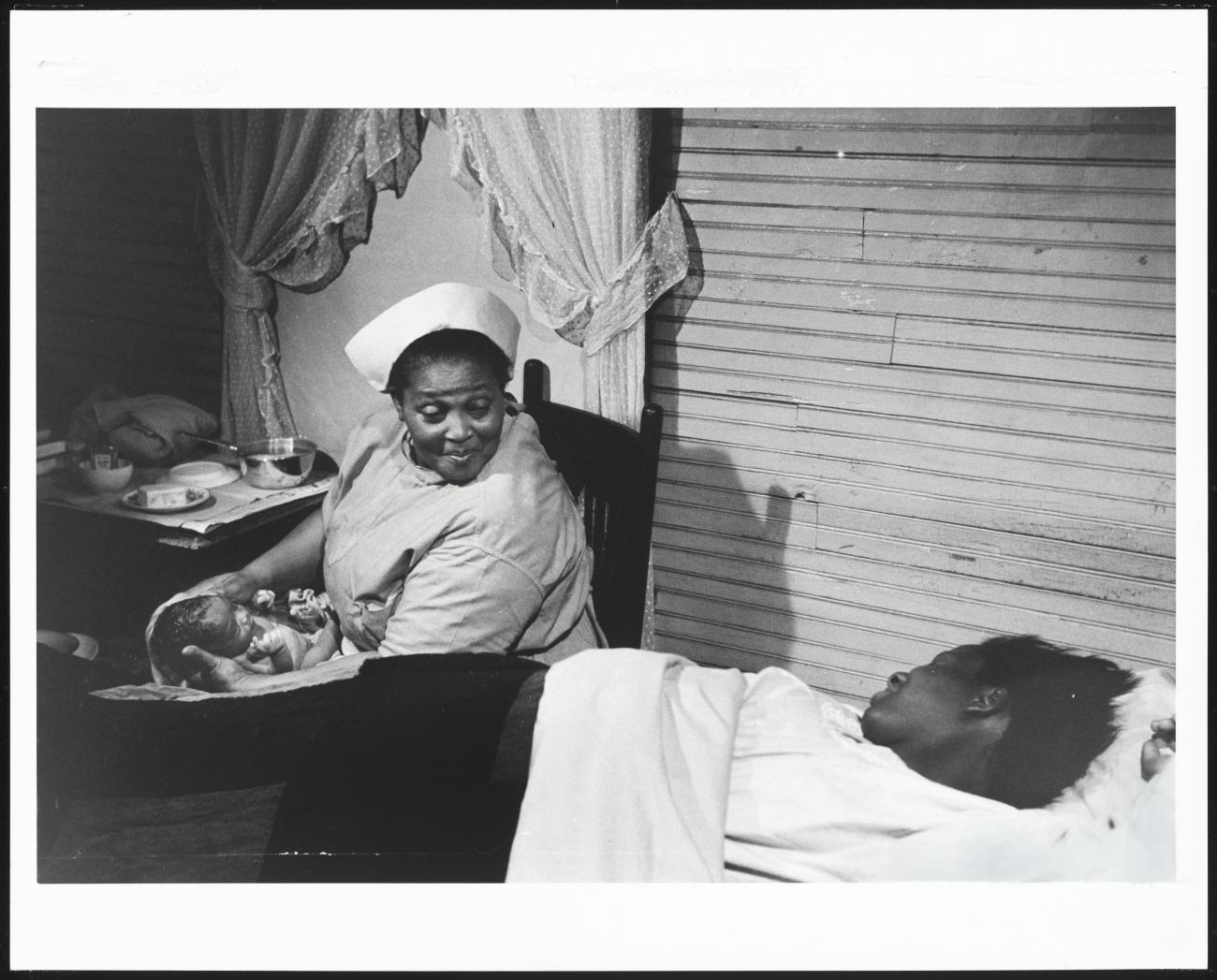This black and white photograph, likely from the 1950s or 60s and often seen in educational materials, depicts a tender post-birth scene with two African women, possibly African American. The woman lying in bed under a series of blankets, with her head pillowed to the right of the frame, gazes down at another woman dressed in a nurse's uniform with a white cap. The nurse, seated in a dark wooden chair to the left of the bed, gently holds and cleans a newborn baby. The background features wooden slats and vintage-style lace curtains, lending an air of nostalgia to the photo. A table with bowls is visible, suggesting post-birth care activities. The walls, reminiscent of paneled garage doors, further affirm the era of the image. The photograph is framed by a white border and a thin black rectangular border, emphasizing its dated authenticity and historic value. The serene, intimate moment beautifully captures the joy and care surrounding childbirth in a less affluent setting from a bygone era.